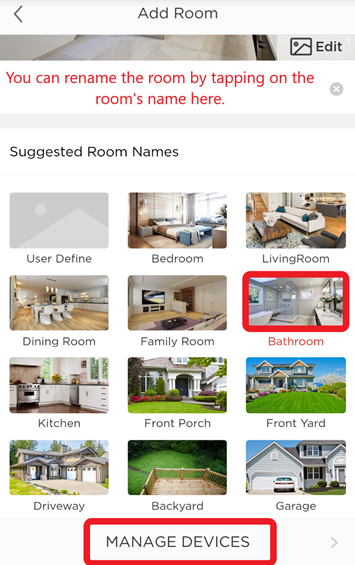The screenshot captures a cell phone interface for adding a room to a home management app. At the top, a light gray horizontal rectangle features a black arrow pointing left, resembling a sideways "V," next to the centered black text "Add Room." Below this title, there is another horizontal rectangle showing a birds-eye view of a small section of a cream-colored tile floor with white walls.

To the right, another rectangle displays a gray background with a square dot in the upper-left corner. Crossing diagonally from the lower left to the upper right and then off the screen, a line is visible. Next to it, the word "Edit" is displayed. Below in red text, it reads: "You can rename the room by tapping on the room's name here."

Further down, a thin gray horizontal rectangle separates the page, and "Suggested Room Names" appears in black text two lines below. The suggestions are organized in four rows, each containing three images. The categories are as follows:

- First row: User Defined, Bedroom, Living Room
- Second row: Dining Room, Family Room, Bathroom (outlined in thick red)
- Third row: Kitchen, Front Porch, Front Yard
- Fourth row: Driveway, Backyard, Garage

At the bottom center, "Manage Devices" is presented in gray all-caps text, enclosed by a thick red rectangle, indicating an interactive element.